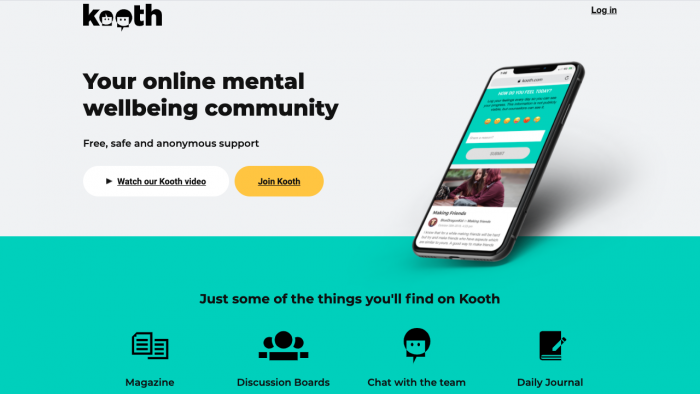The image showcases the homepage of the KOOTH website, a vibrant and user-friendly platform dedicated to mental well-being. The design is striking, with the top half of the webpage featuring a soothing grayish-white background, and the bottom half adorned in a captivating turquoise color.

At the center of the image, a smartphone screen displays the KOOTH website, emphasizing its accessibility on mobile devices. Smiley face emojis are visible, symbolizing the positive and supportive atmosphere of the community. Additionally, there are illustrations of two individuals possibly engaged with content in the background, suggesting a sense of interaction and community.

Distinctive touches include the KOOTH logo, with the 'O's designed as white square boxes with two small black eyes, adding a playful and inviting element to the brand's identity. The tagline "Your online mental well-being community" is prominently displayed in black text, reinforcing the purpose of the site.

The website offers an array of features to support users, highlighted in the turquoise section: "Just some of the things you'll find on KOOTH - Magazine, Discussion Boards, Chat with the Team, and Daily Journal," each accompanied by individual icons representing these services.

Key call-to-action buttons are also visible: an all-white button inviting users to watch a KOOTH video and an orange button encouraging them to join the community. At the very top of the page, there is a "Login" option in black text, allowing existing users to access their accounts easily.

Overall, the image captures the welcoming and resource-rich environment of KOOTH, appealing to users seeking a secure and anonymous space for mental well-being support.